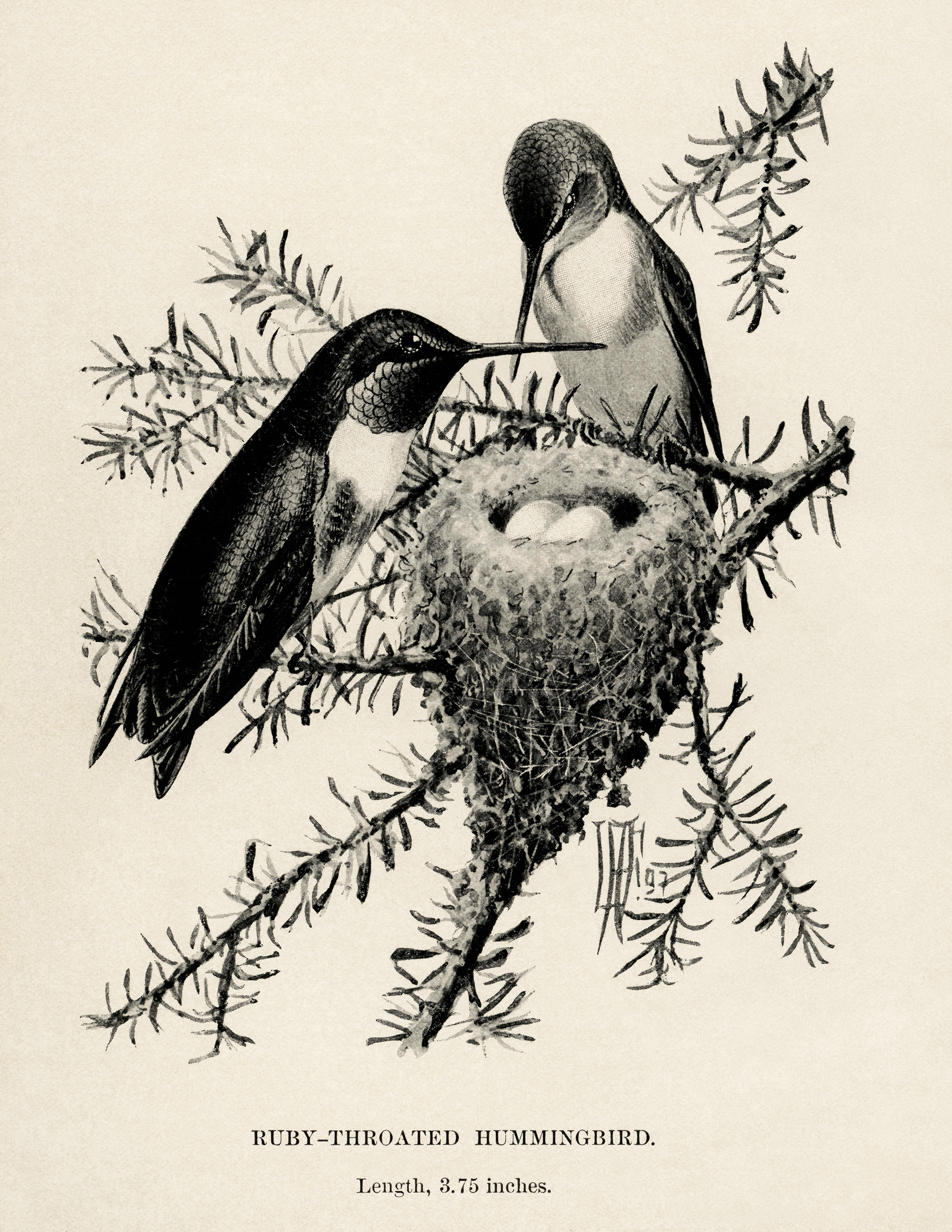This detailed black-and-white drawing, set on ivory cream paper, captures two ruby-throated hummingbirds perched on a branch beside their conical nest, which holds two tiny eggs. The birds, distinguishable by their distinctive long, pointed beaks, are depicted in fine detail: one bird, viewed from the side, showcases a dark back and a white underbelly, while the other bird, facing forward, mirrors this coloration. Surrounding the birds are branches adorned with delicate, pine needle-like leaves. Below the nest, centrally located in the drawing, the artist's signature is visible. Typed text at the bottom of the image identifies the species and provides a measurement: "Ruby-throated Hummingbird, length 3.75 inches." The entire composition rests against a gray background, typical of illustrations found in ornithological books, emphasizing both the artistry and the scientific nature of the piece.